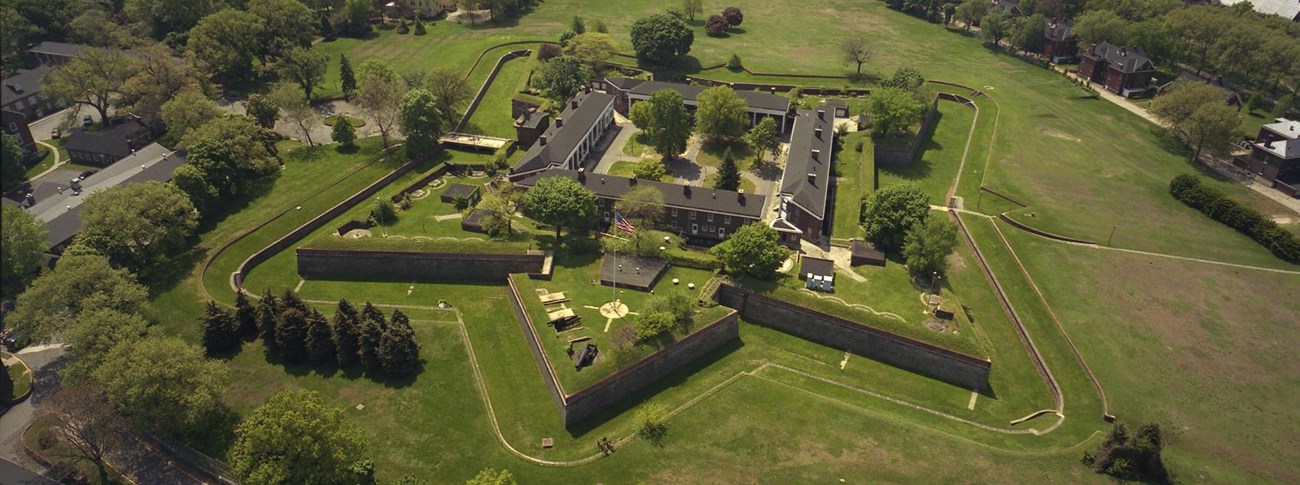Aerial view of an estate with intricate landscaping, captured from a high vantage point. At the center of the image is a square formation of buildings, possibly an apartment complex, featuring a central courtyard adorned with trees and pathways. Surrounding this central structure is a star-shaped design outlined by grass, contributing to the estate's geometric and aesthetically pleasing appearance. The outer edge of the star consists of neatly mowed lawns, additional trees, and smaller structures. To the left, there's a road and an array of houses interspersed with trees, while the right side reveals a mix of fields and more residential buildings. A prominent feature within this scene is a flagpole with an American flag, adding a touch of character to the landscape.